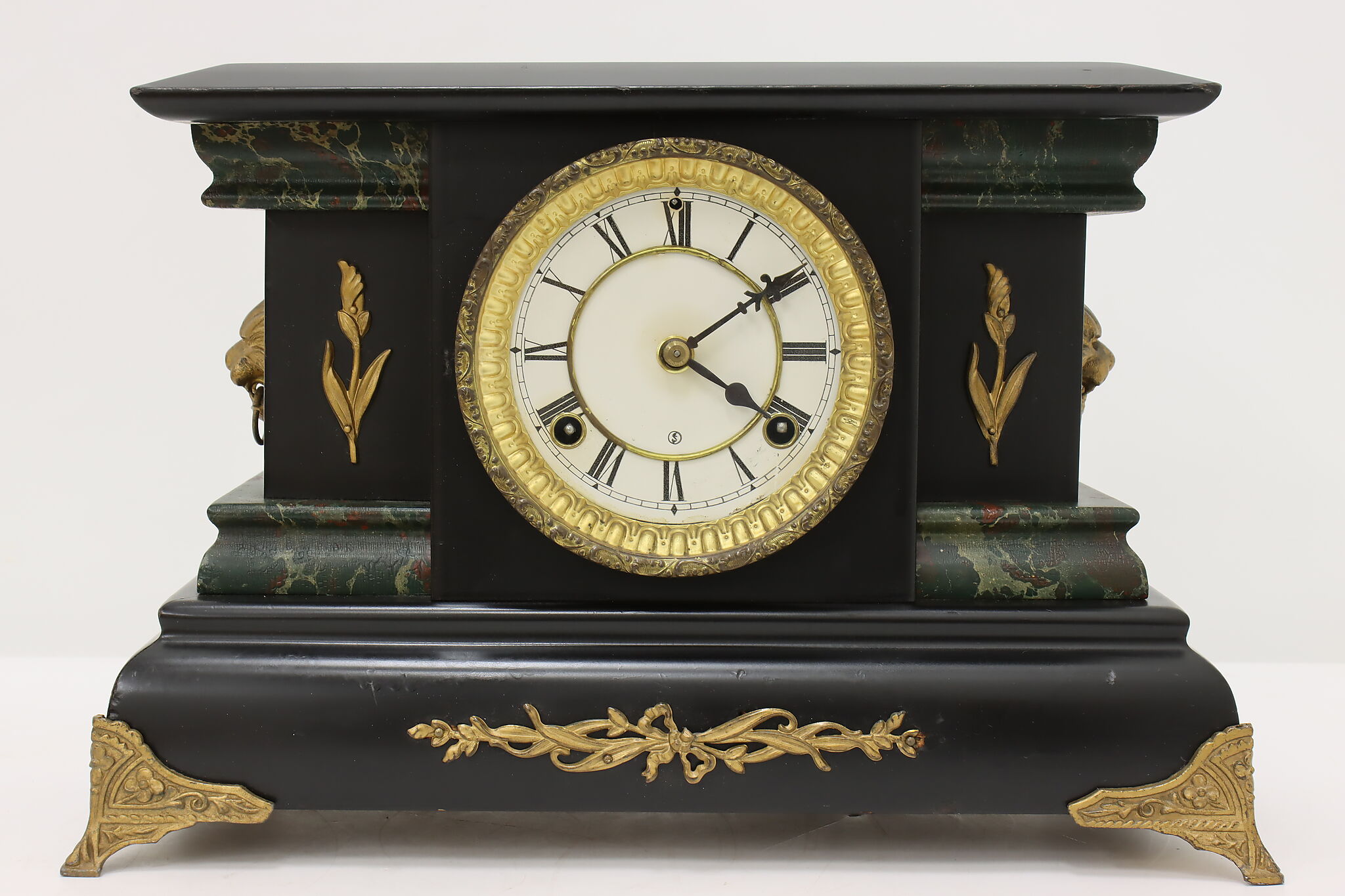This photograph captures an antique wooden clock, exuding a sense of historical elegance. The clock features a circular face accentuated by a gold ring around the dial, with black Roman numerals set against a white background, indicating the time of 3:10. Two small holes are visible near the four and eight o'clock positions, likely entry points for keys to adjust the clock's mechanisms or alarm. The structure encasing the clock is a rectangular black painted wood, complemented by intricate beige-bronze metal feet that angle slightly outward. 

Adorning the sides of the clock face are ornamental gold leaf flowery designs, extending further to form patterns on the feet. Topping the structure, reminiscent of crown molding, is a dark greenish-gray marble-like slab. Additionally, animal head motifs, possibly lions or dragons, embellish each side of the clock, each with a small ring hanging from their mouths, akin to miniature door knockers. The overall ornate design, coupled with the clock's robust build, suggests that it would be an impressive piece to display on a cupboard or in a museum gallery, emphasizing its antique value.